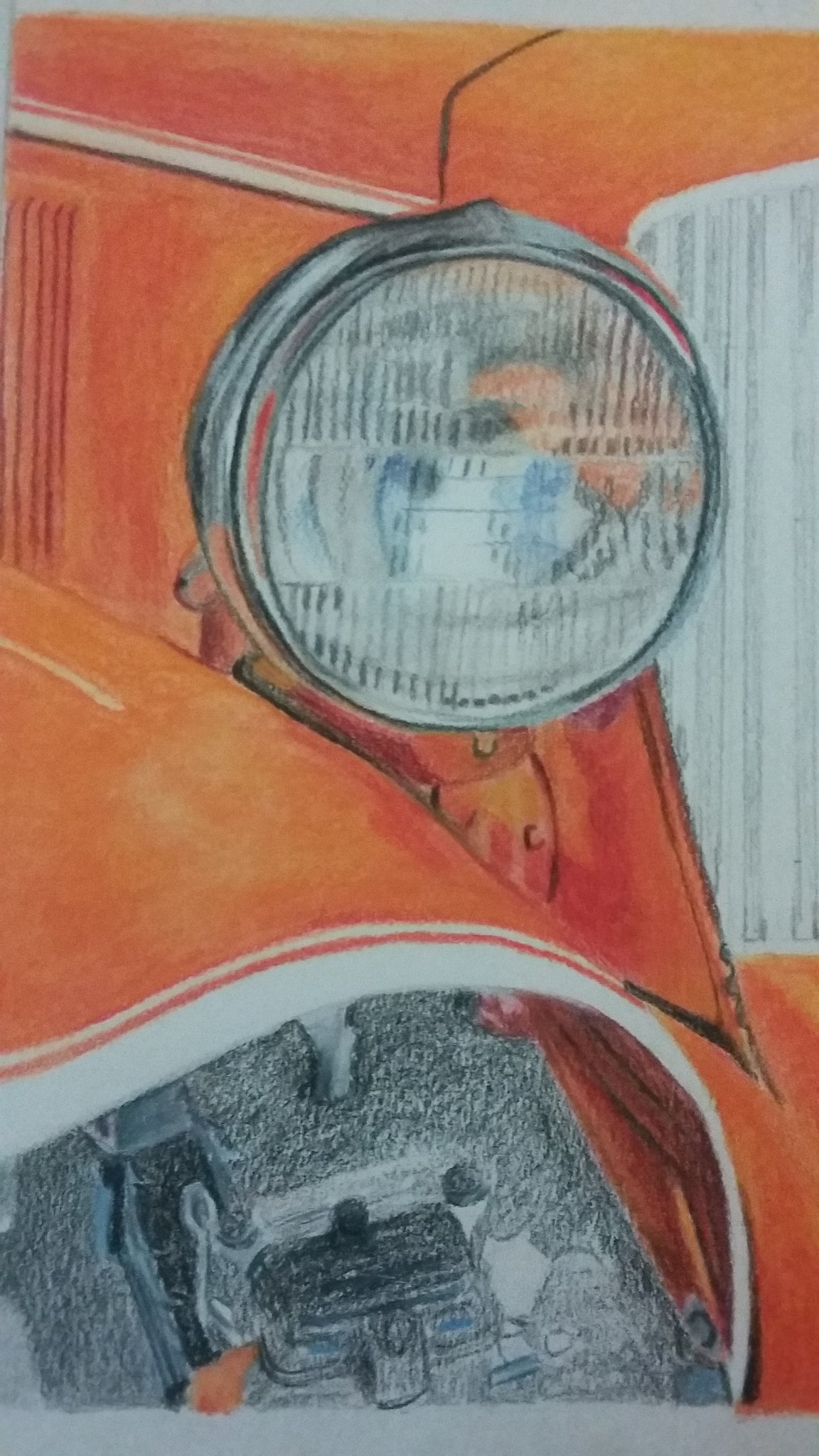A detailed, hand-drawn illustration showcases a close-up section of the front left area of an older vehicle, reminiscent of a classic car from the 1960s. The frame of the car is painted a light, watercolor red. Prominently featured is a circular headlight with a chrome frame, reflecting the distinctive design of that era. The grill beneath the headlight consists of long, vertical white slits. The illustration reveals some of the internal mechanics, possibly the engine, rendered in crayon or colored pencil on textured paper, enhancing the artwork's detailed and tactile feel.